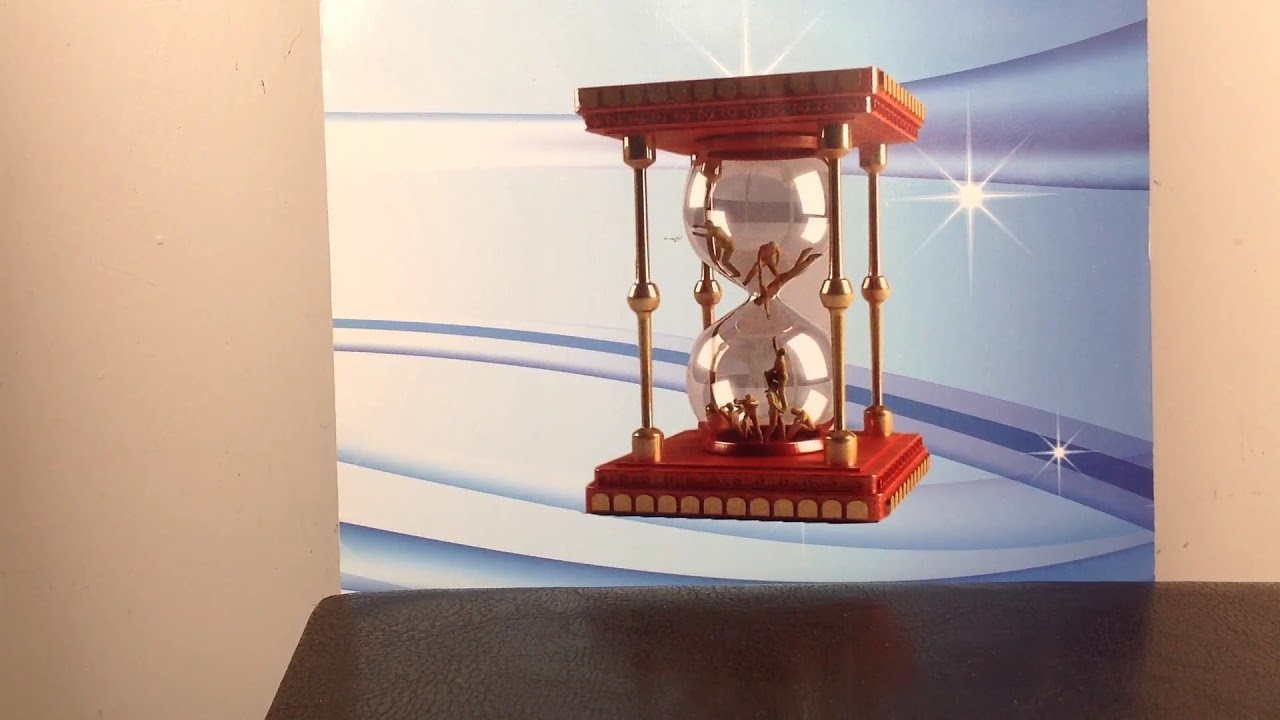The image is a detailed digital artwork featuring an intricately designed hourglass set against a gradient background with waves of blue and purple. The backdrop is adorned with digital star designs, enhancing the cosmic feel of the artwork. The scene appears to be part of a larger painting, possibly photographed, and is placed against a light pink or off-white wall that looks slightly dirty in some parts. Below the painting, there is a surface that resembles either a brown tabletop or a textured desk, possibly with a crocodile or snakeskin pattern. The hourglass itself is framed by a wooden top and bottom with gold metal pillars at each corner. Inside the hourglass, various human-like figures are depicted. Some figures appear to be climbing upward, while others seem to be sliding down, creating a dynamic visual narrative within the confines of the hourglass.